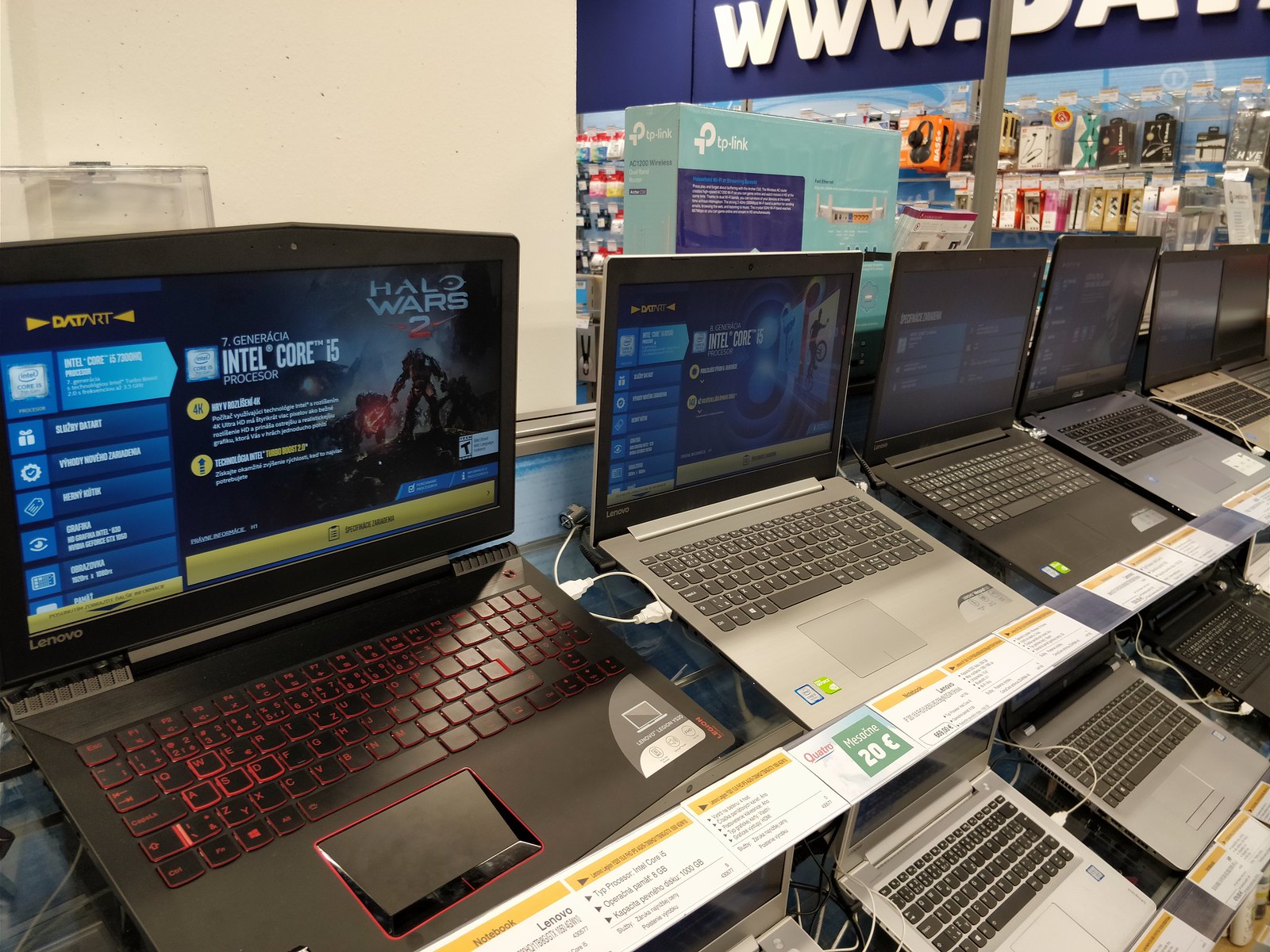The image shows a detailed store display in what appears to be an electronics store, possibly a Best Buy. Prominently displayed are multiple laptops arranged neatly on shelves, organized into two rows. The top row features a striking black Lenovo laptop with red backlit keys, showcasing the game Halo Wars 2 on its screen, along with a brief breakdown of its components. To the right, the displayed laptops alternate between black and silver, with the silver ones lacking backlit keyboards. Above these laptops is a boxed TP-Link router, recognizable by its blue packaging and white router with yellow Ethernet ports. In the background, a variety of electronics accessories and supplies hang on brackets, including headphones. The scene is anchored by a blue wall with a partially visible sign in giant white letters that reads "WWW dot." This immersive setup effectively showcases the products, inviting customers to explore the different laptop models and their features.